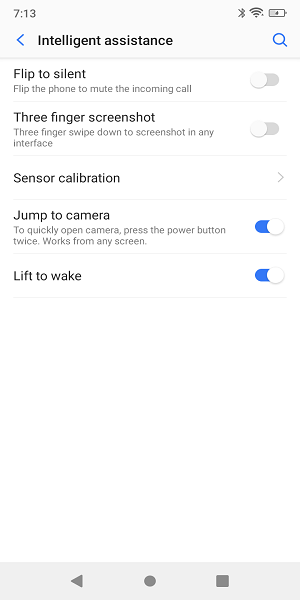The vertical rectangular screenshot captures a smartphone interface within a specific application page. At the top of the screen, the time is displayed as "7:13" in the left corner. In the upper right corner, icons for Bluetooth, Wi-Fi, and battery status are aligned in sequence. 

Directly below, on the left side, a blue back arrow is visible, leading the section headers. To its right, the title "Intelligent Assistance" is prominently showcased in bold black text, with a search icon adjacent to it on the far right.

The content beneath this header presents several selectable options, each accompanied by a toggle switch on the right. The first option is "Flip to Silent," which allows the user to mute incoming calls by flipping the phone; its toggle is currently off. The next option, "Three-Finger Screenshot," which captures the screen using a three-finger gesture, is also toggled off.

Further down, "Sensor Calibration" is listed with an arrow on the right side indicating the possibility to delve deeper into its settings. Following this, "Jump to Camera," which quickly opens the camera by pressing the power button twice regardless of the current screen, has its toggle switched on. Lastly, "Lift to Wake," a feature that wakes the phone when picked up, is shown as activated, with its toggle in the on position.